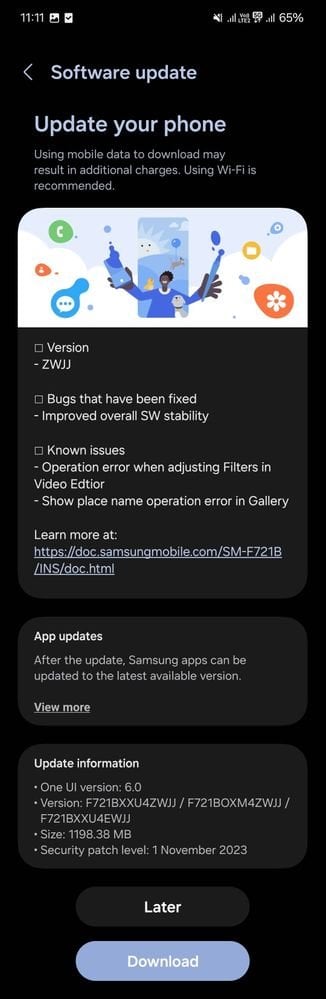A vertically-oriented image captured from a cell phone screen displaying a software update notification is shown. The image appears slightly distorted, having been squished vertically. The backdrop is solid black. In the upper left corner, a timestamp reads "11:11," accompanied by two icons. Moving to the upper right, there's an array of five mobile signal icons alongside a battery indicator displaying "65%."

The primary focus of the screen is the software update notification, suggesting that using mobile data for the download may incur additional charges and recommending Wi-Fi usage. Importantly, the image suggests this is a non-iPhone device, likely a Samsung, as inferred from the specific language in the notification and the mention of Samsung apps.

An icon featuring a person holding two objects, potentially a phone and a microphone, appears, indicating engagement or interaction with the device. Below this, detailed information about the software update is presented:
- Download version: ZWJJ
- Fixed bugs: Enhanced overall software stability
- Known issues: Information available at appupdates

Further clarification mentions post-update Samsung app updates, reinforcing the device type. Additionally, specifics of the update include "One UI version 6.0" and a long version string. At the bottom of the screen, two buttons offer the user options to "Later" delay the update or "Download" to proceed with it.